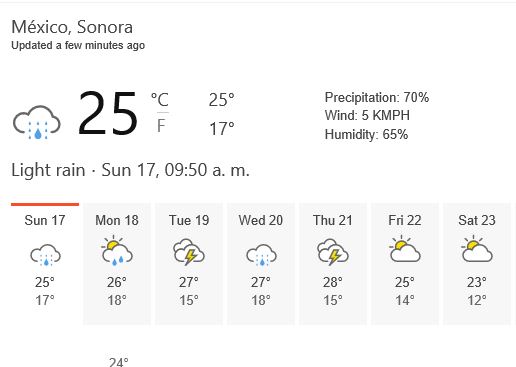A detailed screen capture of a weather forecast for Sonora, Mexico, updated a few minutes ago. The forecast spans the upcoming week, displaying temperatures in Celsius over a white background with black text. Symbols denote light rain and thunderstorms, with light rain specifically indicated for Sunday the 17th at 9:50 a.m. 

Currently, the temperature is 25°C with 70% precipitation, 5 km/h winds, and 65% humidity. 

The forecast details are as follows:
- **Sunday, 17th**: High of 25°C, Low of 17°C, Light Rain.
- **Monday, 18th**: High of 26°C, Low of 18°C.
- **Tuesday, 19th**: High of 27°C, Low of 15°C, Cloudy with possible thunderstorms.
- **Wednesday, 20th**: High of 27°C, Low of 18°C.
- **Thursday, 21st**: High of 28°C, Low of 15°C.
- **Friday, 22nd**: High of 25°C, Low of 14°C.
- **Saturday, 23rd**: High of 23°C, Low of 12°C.

At the bottom of the chart, there's a partially visible text showing 24 degrees which is incomplete.